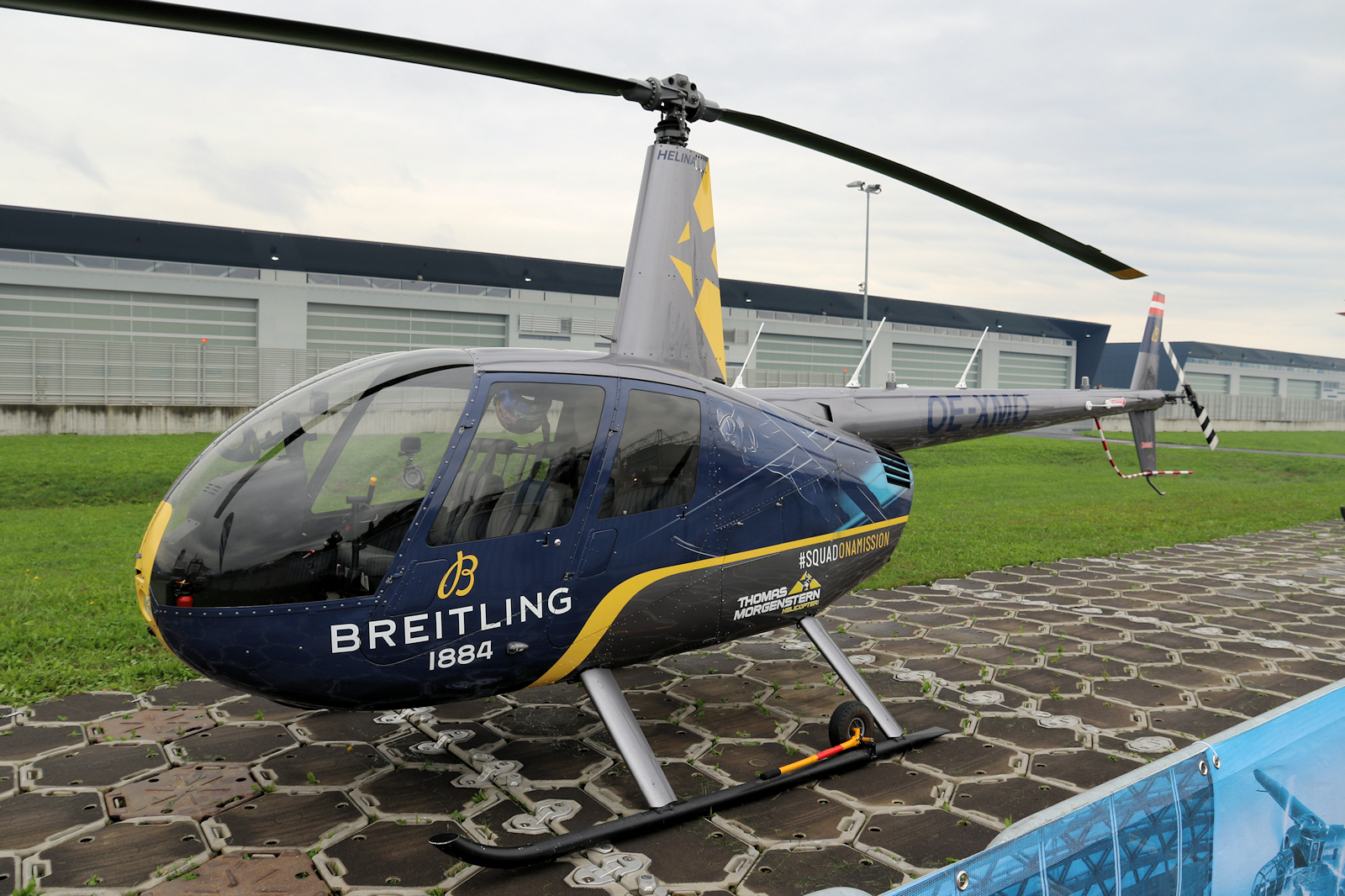The image features a navy blue, yellow, gray, and black helicopter prominently centered, slightly off-center to the left. The helicopter is bulbous and oval-shaped, with glass windows on the front and sides, resembling an egg. It has silver legs and a ski-like bottom. Displayed on the helicopter are the words "Breitling 1884" in uppercase white letters near the door, with a yellow "B" above "Breitling". Toward the rear, it reads "#squad on a mission" and "Thomas Morgenstern" in capital letters, along with a yellow logo. The tail section is marked with "D-E-X-M-D".

The helicopter is situated on a black pavement with yellow and white circles. Surrounding the scene is a concrete path of brown and gray hues. In the background, there is a stretch of light green grass, beyond which lies a row of warehouse sheds made of silver metal and black roofs. Above, the sky occupies the top quarter of the image, displaying a cloudy, light blue expanse.